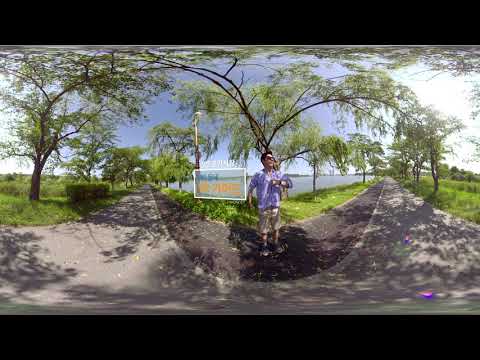The image depicts an outdoor scene, likely taken in the midst of a public park on a sunny day. The setting is framed by a solid black border at the top and bottom. At the center of the image stands a man with short dark hair and sunglasses, dressed in a blue short-sleeved shirt and tan shorts. His footwear could either be roller skates or running shoes. He is positioned on an asphalt pathway or at the intersection of two converging roads, which creates a gray, upside-down rainbow effect around him. Surrounding him is a grassy landscape dotted with trees that have thin branches and leaves extending outward, casting shade over the man.

In the background, directly behind the man, there's a wedge of greenery flanked by trees, stretching out into the horizon where a body of water and some faint building structures can be seen. To his right, over his shoulder, there is a sign with orange lettering, though the text is unclear. The sky above is adorned with a blend of blue and white, adding a tranquil backdrop to this serene park setting. The scene is rich in colors, including black, gray, green, purple, orange, and dark blue, giving depth and vibrancy to the photo.